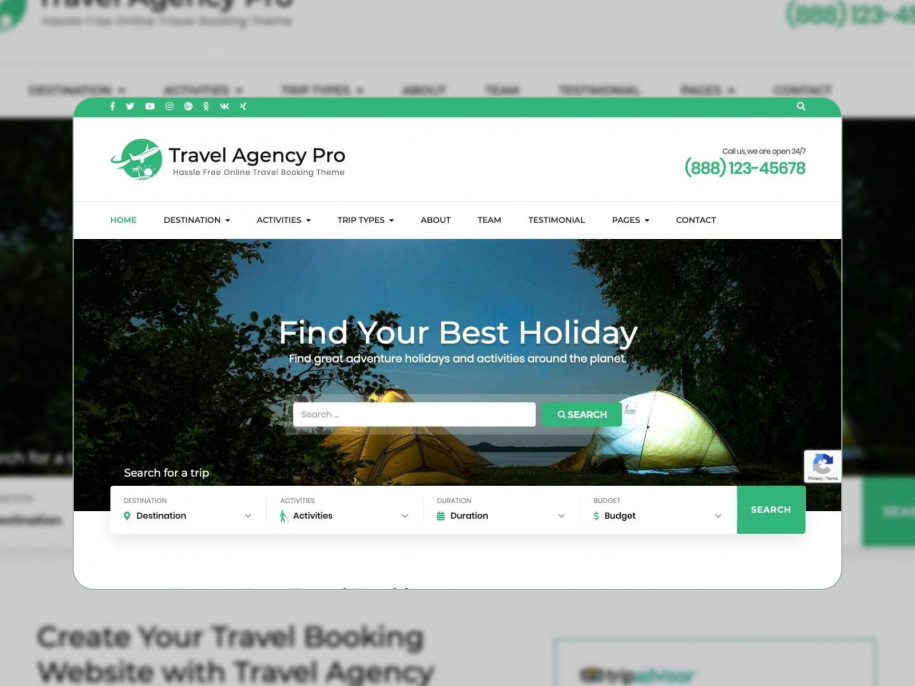This image is a screenshot taken from a website named "Travel Agency Pro." The full website interface is visible in the background, but a prominently placed popup box invites users to "Find Your Best Holiday."

The website features a green icon showing an airplane, a palm tree, and a sun, emphasizing a hassle-free online travel booking experience. The main navigation bar includes dropdown options for Home, Destination, Activities, Trip Types, About, Team, Testimonial, Pages, and Contact.

At the top of the page, there's a prompt urging users to "Call us, we are open 24/7," with a green-highlighted phone number (888) 123-45678.

The central popup box is designed for users to effortlessly plan their next holiday. It reads, "Find Your Best Holiday" and below, it encourages finding "Great Adventure Holidays and Activities Around the Planet." Users can enter their preferences in a search box featuring various criteria such as Destination, Activities, Duration, and Budget. To ensure safety, a CAPTCHA verification step is included before initiating the search via a button with a magnifying glass icon labeled "Search."